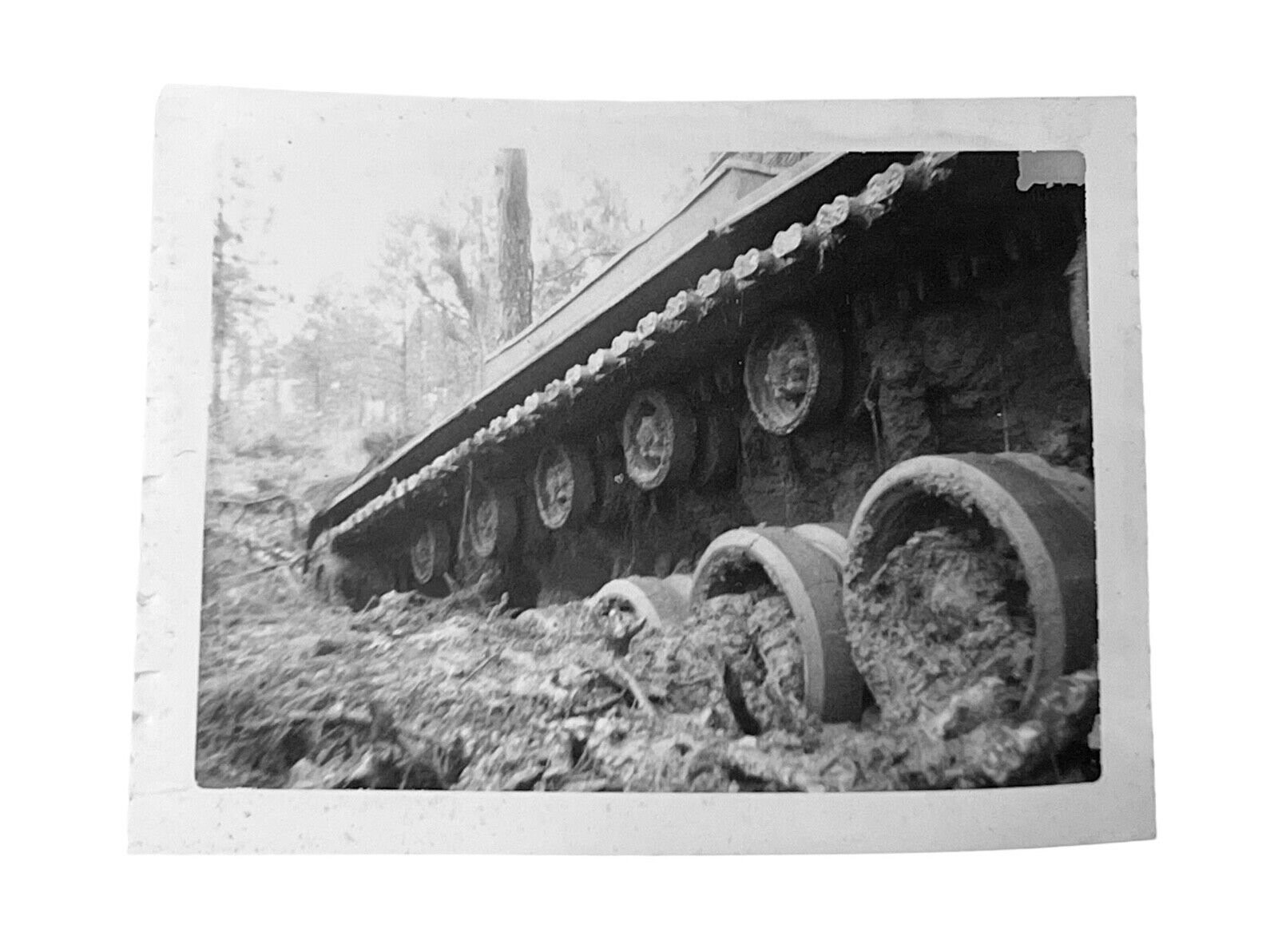This is a black-and-white photograph, aged and curling, with a light gray border that fades into the picture at the top left corner, becoming darker towards the right. The image, approximately five inches wide and three inches high, features a muddy outdoor scene that appears chaotic. Central to the composition are the tracks and wheels of a military vehicle, possibly a tank, either emerging from or sinking into a hill of thick mud. The cylindrical tank wheels, aligned in a row, are heavily caked with mud, blending into the muddy background. The muddy terrain envelops the lower portion of the tank, suggesting a struggle through difficult terrain. In the background, there are sparse trees and brush, adding to the desolate and messy appearance of the scene. The photograph lacks visible borders and seems to have been taken from a low angle, emphasizing the challenging conditions faced by the vehicle.